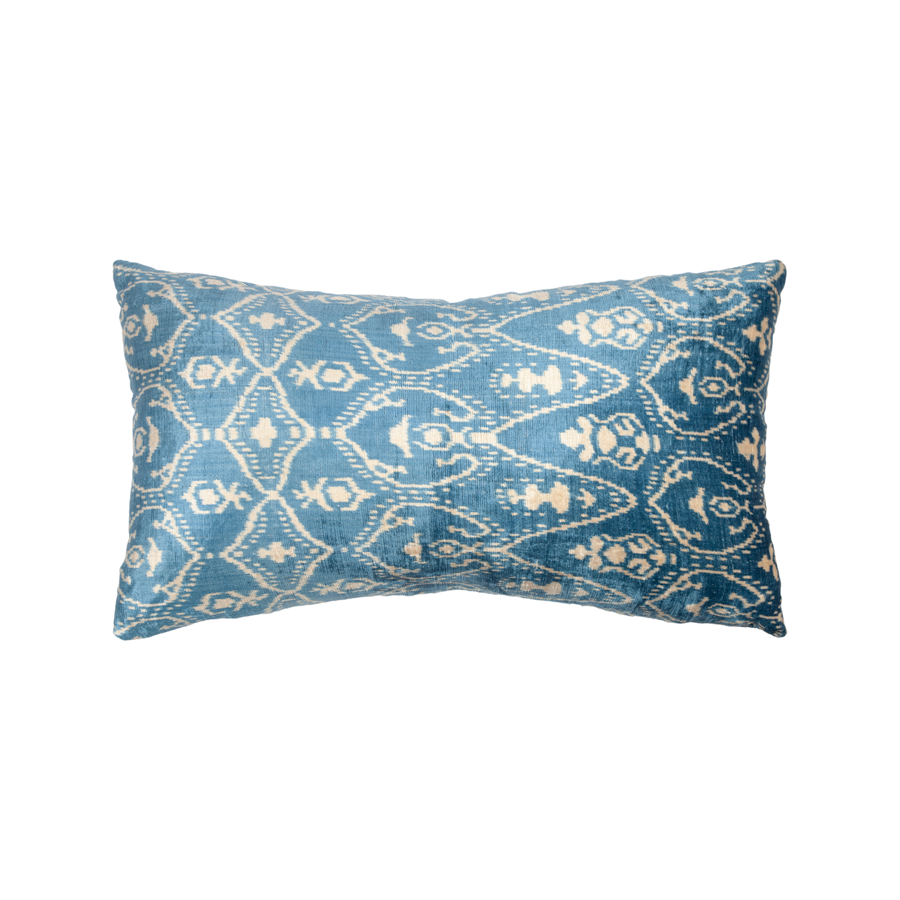The image depicts a rectangular throw pillow, possibly intended for a couch, adorned with ornate patterns. It is blue with intricate off-white, beige, or accrue designs, reminiscent of Mediterranean, North African, or Middle Eastern motifs. The pattern features repeated semicircles and curved lines, which create a traditional, non-European aesthetic. Elements of Damask-like designs suggest a Victorian influence, adding to its intricate and elegant appearance. The pillow is presented against a bright white background, emphasizing its detailed blue and white patterns, which appear to be drawn with fine lines outlining various shapes. The zoomed-in view highlights the vertical rows of circular and curved shapes, making the pillow's elaborate design the focal point.